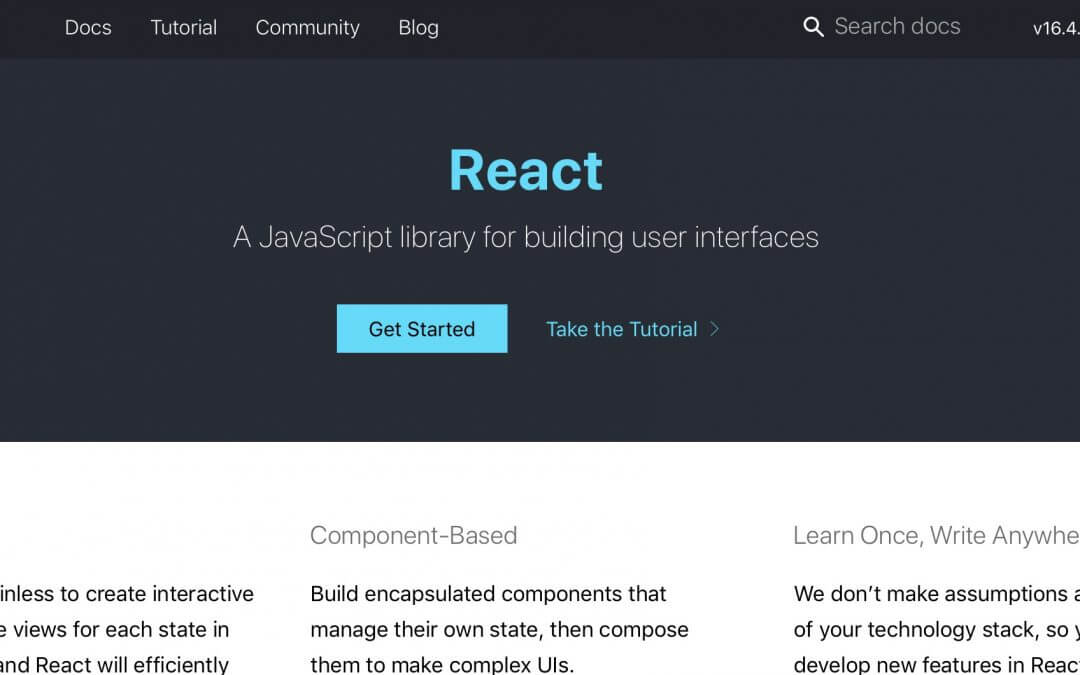The image is a webpage for React, a JavaScript library. The background of the top part of the page is black. In the upper left corner, there are white text links labeled "Docs," "Tutorial," "Community," and "Blog." In the upper right corner, there's a search bar.

In the middle of the page, "React" is displayed in light blue text with the subtitle "A JavaScript library for building user interfaces." 

Beneath this, there is a blue rectangular button with black text that says "Get Started." Next to this button, "Take the Tutorial" is written in blue text.

The background beneath this section is white, with text printed in either gray or black. The text begins with "To create interactive," but some words are cut off. It continues with "Views for each state in," but again, some wording is missing. "React will efficiently" follows.

The next portion describes React as "component-based" with the text, "Build encapsulated components that manage their own state, then compose them to make complex UIs."

The final column, which is partly cut off on the right side, has a header that reads "Learn once, write anywhere," with the initial letters "RE" truncated. The accompanying text states, "We don't make assumptions," but some words are cut off. It concludes with "Develop new features in React."

This summary encapsulates all the textual information present on the webpage.